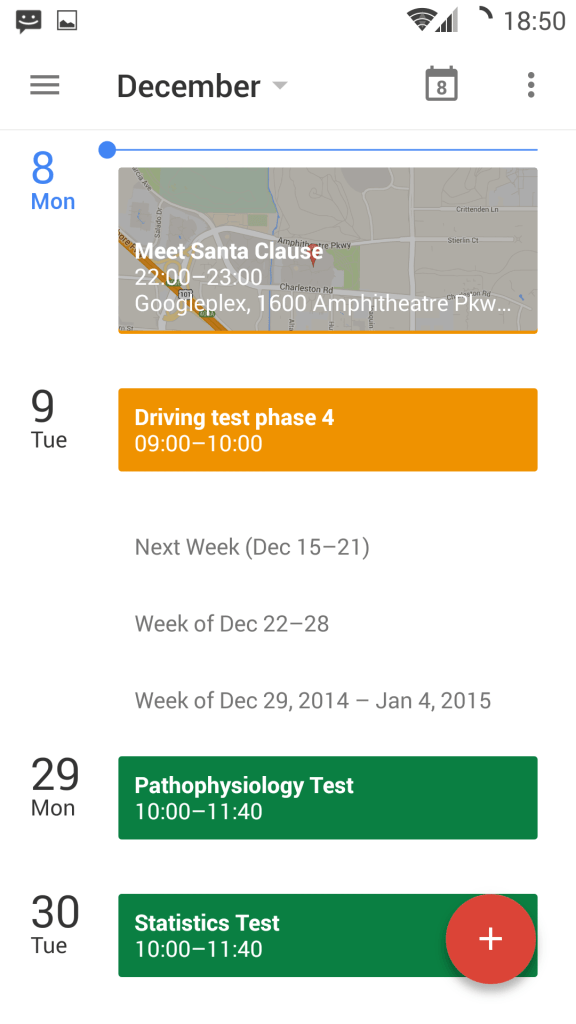The image appears to be a screenshot of a smartphone displaying a calendar or scheduling app interface, set against a predominantly white background. 

At the top of the screen, there is a rectangular notification box featuring a smiley face, possibly indicating the receipt of a new message. Adjacent to this, the status bar shows various symbols, including a gallery icon and a strong Wi-Fi signal with three out of four bars filled, suggesting good reception. The time displayed is 18:50. 

On the left side of the screen, three gray horizontal lines are visible, likely representing a menu icon. Below this, in black text with a capitalized 'D', the month "December" is noted alongside a light gray downward-pointing triangle and the number '8' in gray, indicating the specific day. Further down, there are three gray circles and a thin gray line. 

On the left, the number '8' is highlighted in blue with 'MON' (for Monday) beneath it. A map image is partially covered by white text detailing an event: "Meet Santa Claus, 22:00 - 23:00 at Googleplex, 1600 Amphitheatre Pkwy...".

Immediately below, on the left side, is the number '9' in black with 'TUE' (short for Tuesday) beneath it. An adjacent orange rectangle contains white text announcing another event: "Driving Test Phase, 09:00 - 10:00". Additional scheduling information in gray text mentions upcoming weeks, noting "next week (DEC 15-21)", "week of DEC 22-28", and "week of DEC 29, 2014 - JAN 4, 2015".